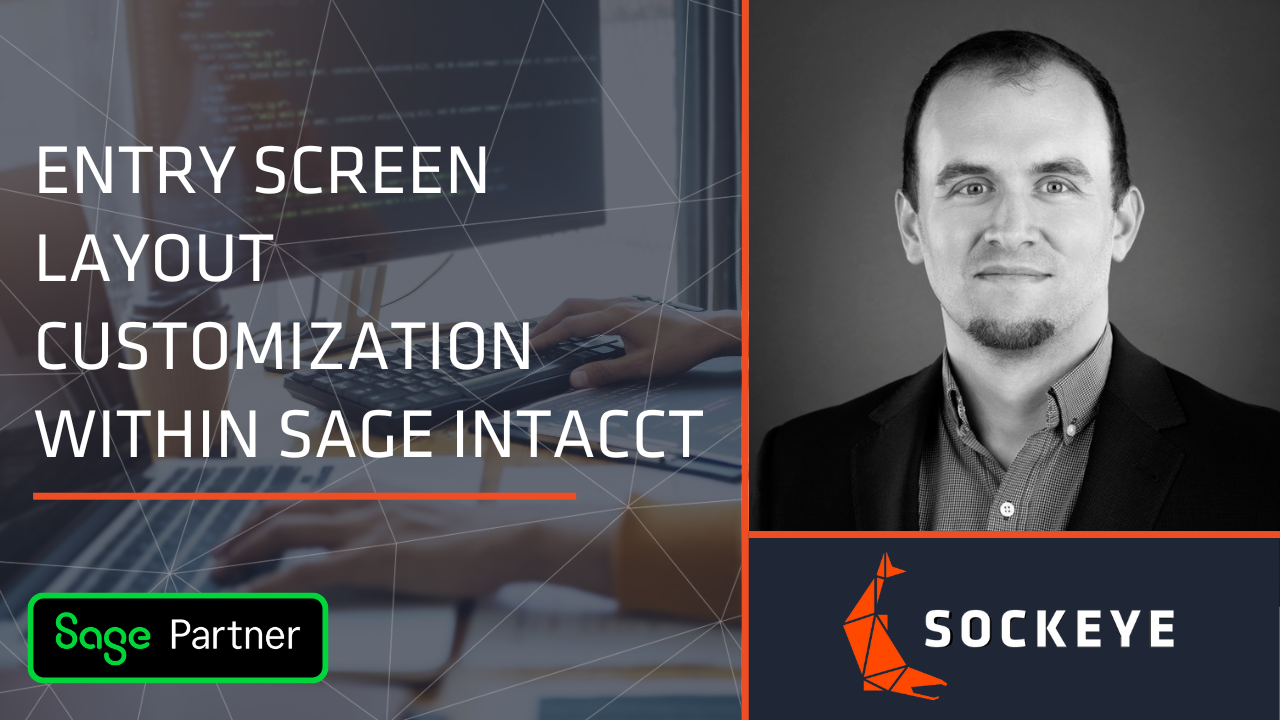The image portrays a dimly lit scene of intense work, with a focus on productivity and technical intricacy. Dominating the visual are a pair of hands typing on two different full-sized keyboards, giving the impression that one person is engaged in a demanding multitasking effort, possibly related to coding or online work. Superimposed over this scene are the words: "Entry, Screen, Layout, Customization, Within, Sage Intacct." Below this text, the branding logos "Sage" and "Partner" are clearly visible. 

To the right side of the image, there is a photo of a man who is slightly balding and sports a chin beard. He is dressed formally in a collared shirt topped with a suit coat or blazer, and he gazes directly at the camera. Below his image, the text "Sockeye" is prominently displayed, possibly referring to a company, brand, or relevant context related to the overall theme of the image.